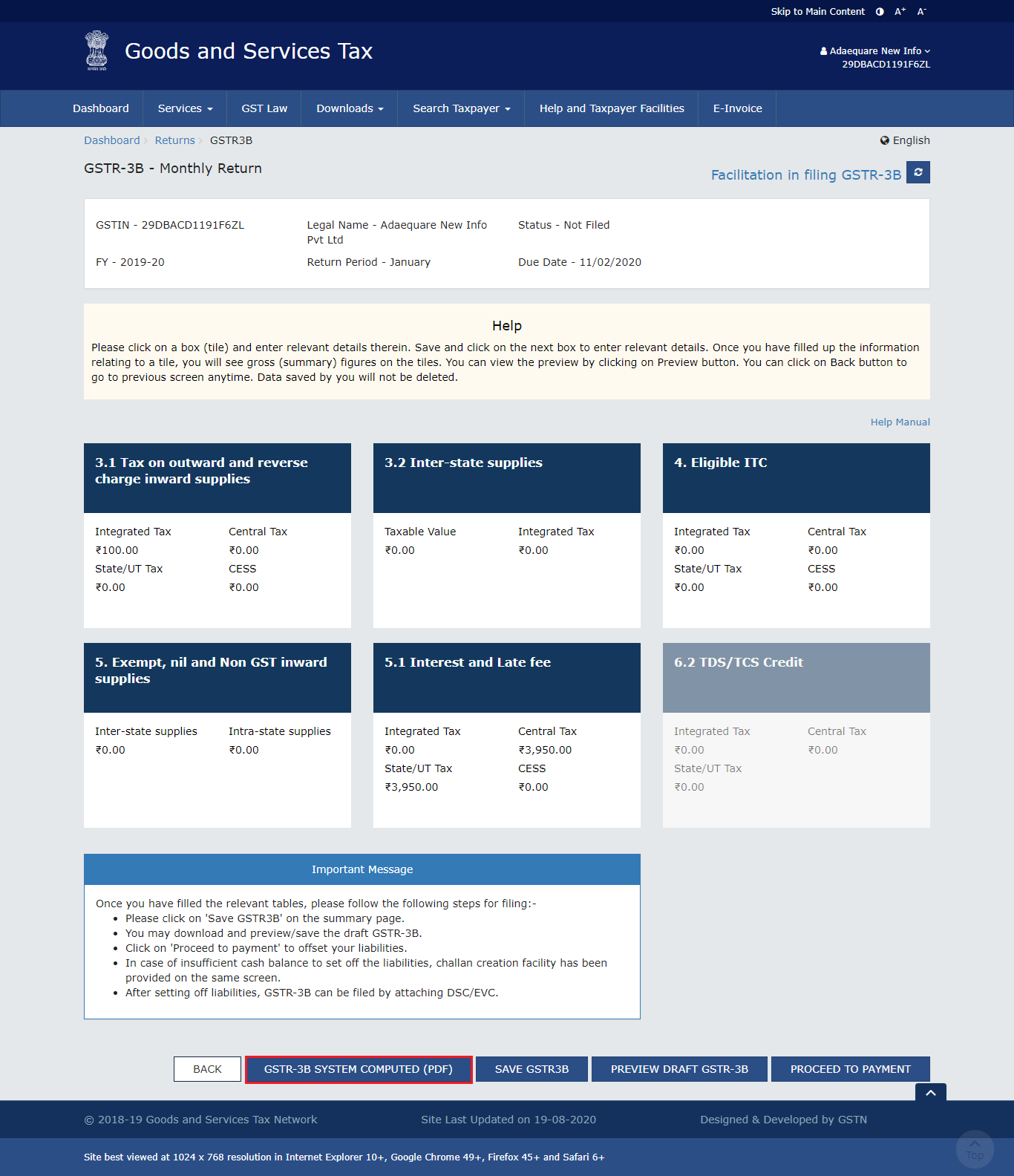This image is a screenshot of a webpage related to the Goods and Services Tax (GST). At the top of the screen, there is a navigation bar with several options, including "Dashboard," "Services," "GST Law," "Downloads," "Search Taxpayer," "Help and Taxpayer Facilities," and "E-Invoice." 

Just below this navigation bar, the title "GSTR-3B Monthly Return" is prominently displayed. The screen also shows a specific account number, the legal name associated with the account, and the current status of the return.

The central part of the screen is predominantly gray, and towards the top, a more prominent ivory-colored box provides instructional text. The instructions read: "Please click on a box tile and enter relevant details therein. Save and click on the next box to enter relevant details. Once you have filled up the information relating to a tile, you will see gross summary figures on the tiles. You can view the preview by clicking on the preview button. You can click on the back button to go to the previous screen at any time. Data saved by you will not be deleted."

Below this instructional box, there are input fields and various boxes where the user can enter details as required. At the bottom of the screen, there are additional options, including "Go Back," "Other GSTR-3B System Computed," "Save GSTR-3B," "Preview Draft GSTR-3B," and "Proceed to Payment."